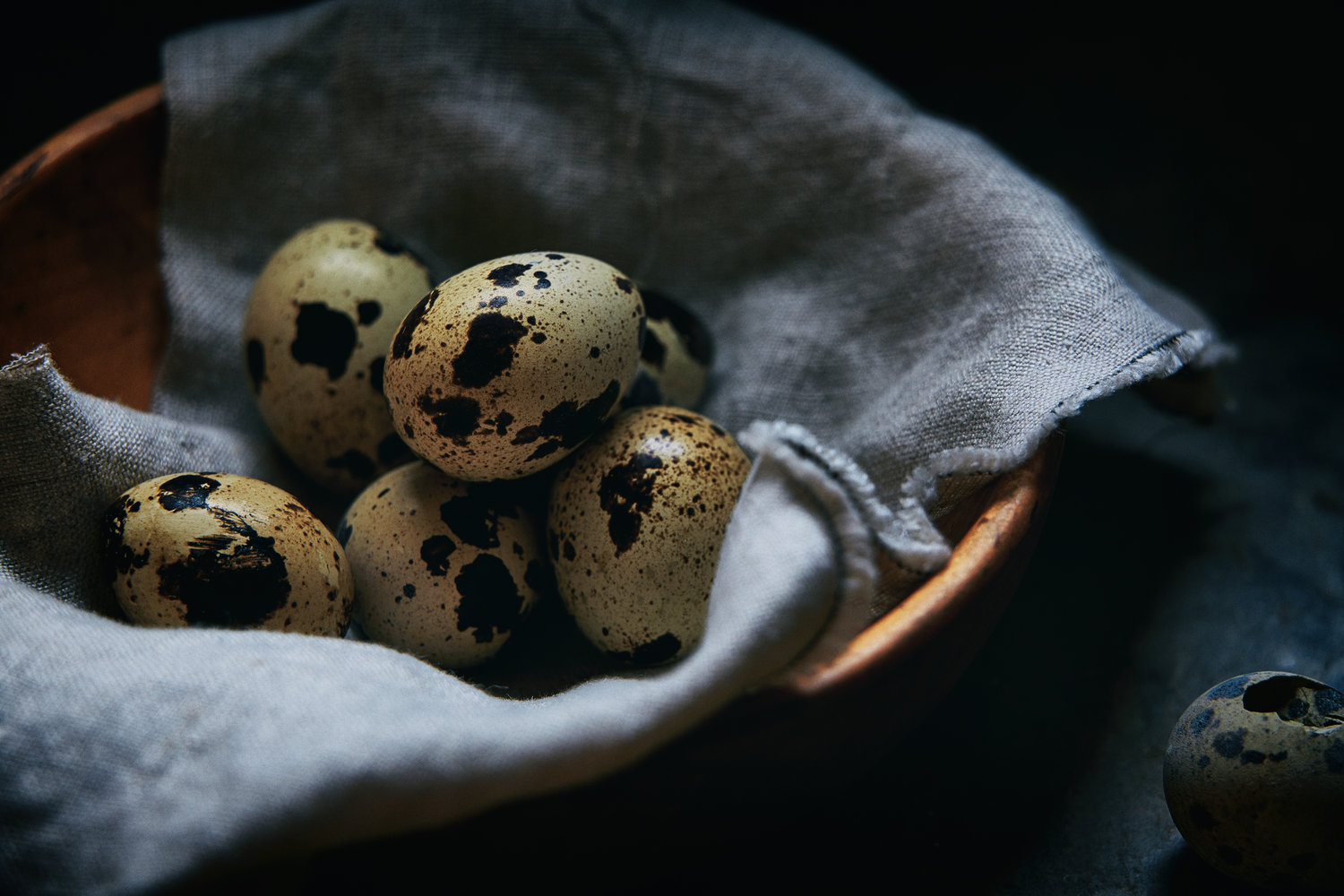The still life photograph features a rustic wooden bowl resting on a dark backdrop. Inside the bowl, a light-colored linen cloth cradles six small, speckled eggs. The eggs, likely robin eggs due to their diminutive size, are primarily white with black and brown speckles in various sizes. One egg is positioned outside of the bowl, showcasing a small crack with a hint of what might be a bird preparing to hatch. The overall lighting is dark and moody, emphasizing the textures and natural beauty of the arrangement.